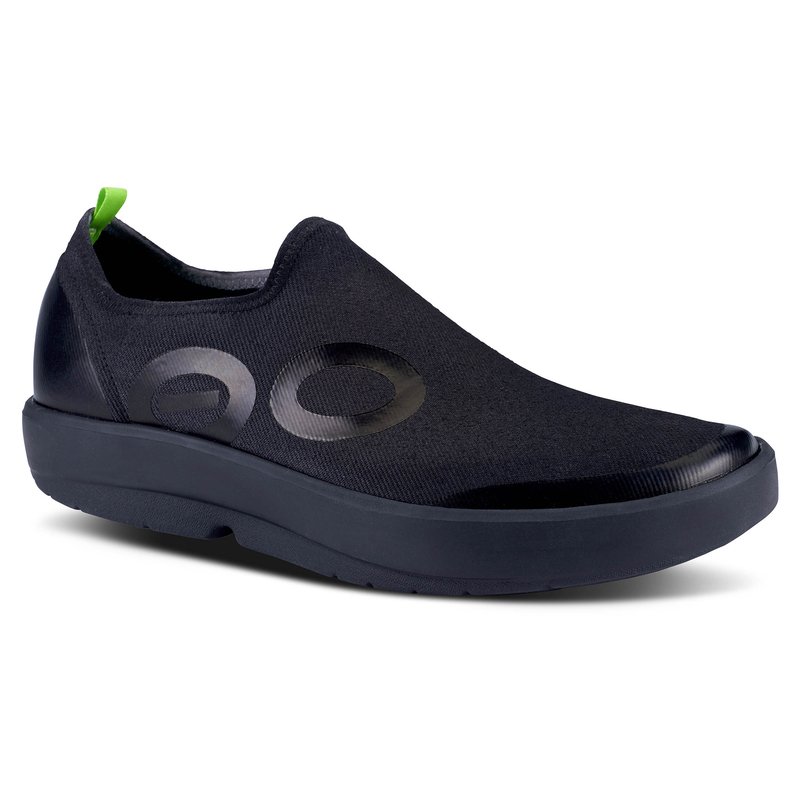This image features a black slip-on shoe, captured from a side profile with the toe facing left. The shoe is set against a white background with a white surface beneath, cast in a slight shadow. The upper part of the shoe is made of a black canvas-like material, contrasted by a black rubber sole which is notably thick and slightly dull in texture. On the side of the shoe, there are two glossy circular decorations resembling flattened O shapes; one of these O's has a line running through it. These decorations are slightly grayer compared to the rest of the shoe. The shoe also features a small, lime green pull tab at the back, designed to help slip the shoe on. Notably, there are no laces, straps, or buttons, as the shoe is a simple slip-on design. The front and back of the shoe feature some shiny black trim, which appears almost plastic-like compared to the canvas-like material.